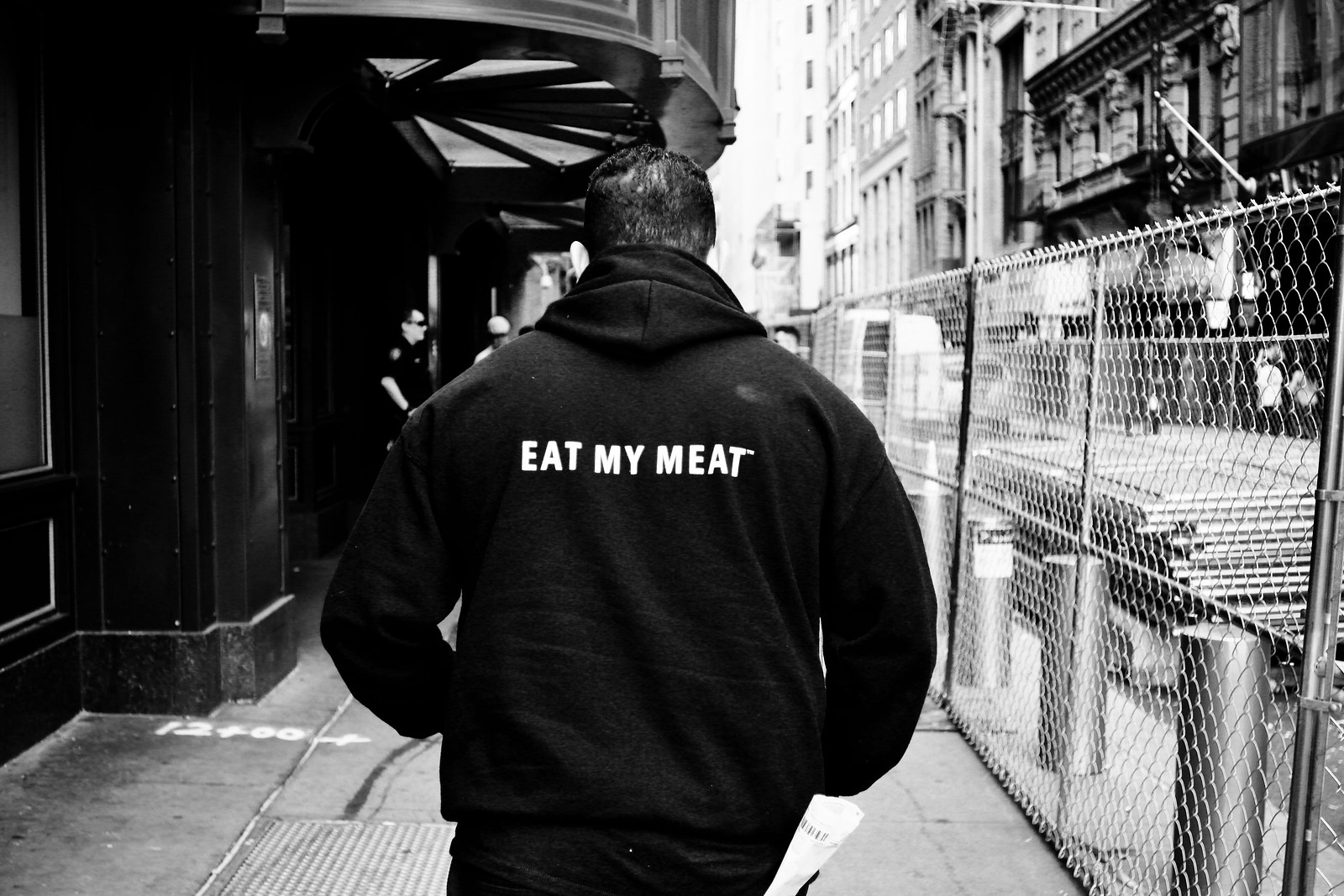In this detailed black-and-white photograph taken outdoors during the daytime in a city, a man is captured walking away from the camera down a gray city sidewalk. The man, who appears to be white with short, dark hair (possibly tied up in a bun), is dressed in a black hoodie with the phrase "Eat My Meat" printed in white letters across the back along with a tiny trademark symbol next to the "T." He also wears dark jeans.

To the left of the sidewalk, there is a line of shops, including a prominent building with a marquee overhanging the sidewalk, which creates an awning area. Beneath this awning, there's a man who looks like a police officer, identifiable by his black shirt with an emblem on the right side and sunglasses, engaging in conversation with another person. 

To the right of the central figure, a chain-link fence runs parallel to the sidewalk, beyond which construction activity is visible, characterized by wooden planks or pallets stacked on a moving structure. Further in the distance on the right side of the image, tall multi-story buildings loom, adding to the urban backdrop. There are a few other individuals visible on the sidewalk ahead of the man, enhancing the bustling city ambiance.